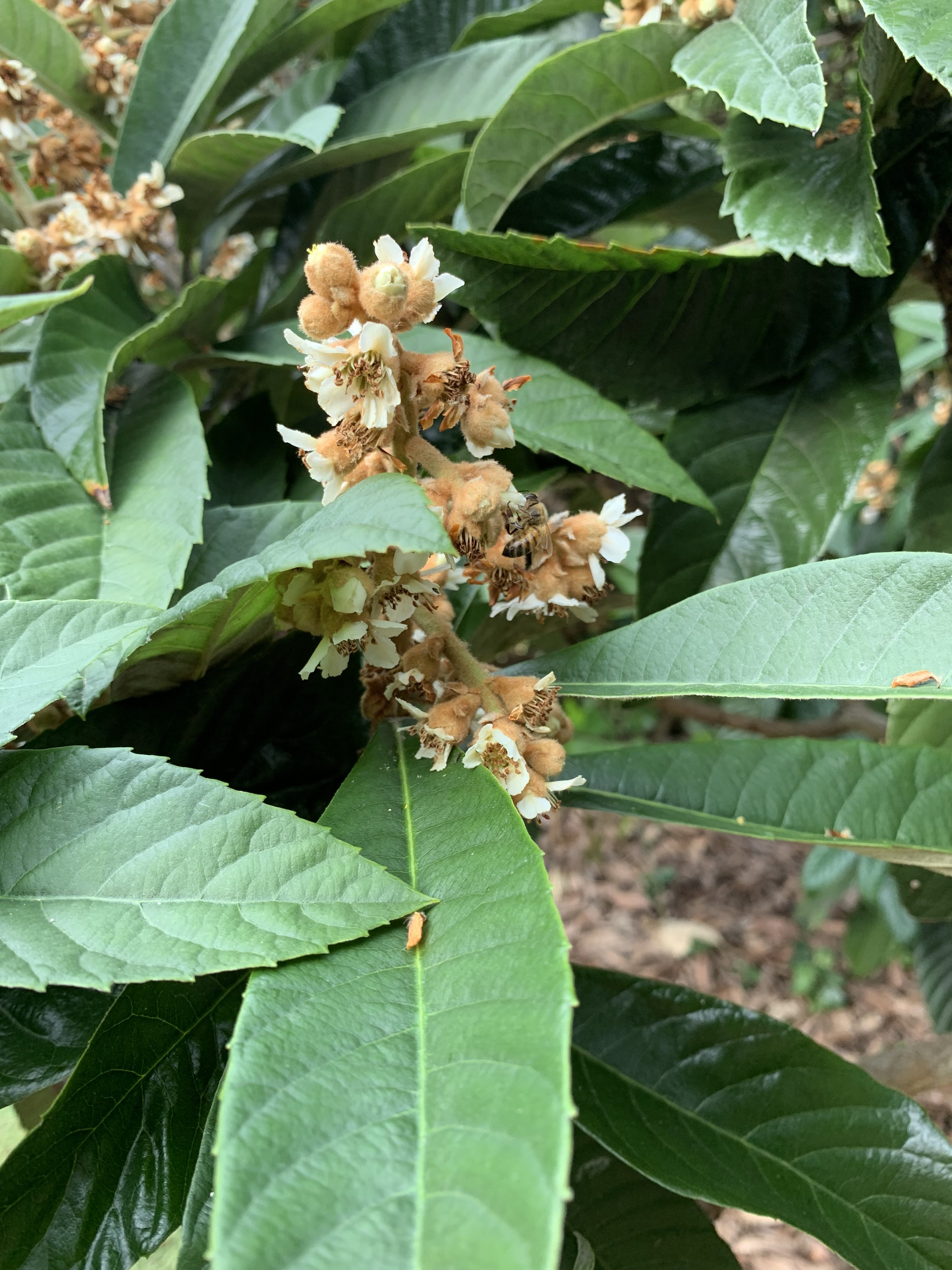This is a close-up photo of a plant or bush taken outdoors, capturing various detailed elements of its flora and surroundings. The plant showcases fronds with differing shades of green, from darker hues on the underside to lighter, almost whitish tones on the top. In the central part of the image, small, blooming flowers stand out; they have white petals with light brown bases and are encircled by numerous stamen and pistils.

Reflecting the late spring season, some of these flowers appear to be nearing the end of their bloom, with parts beginning to fade. Bumblebees are visible on the flowers, attracted to the ones that have already bloomed as they search for nectar, while others rest on the unopened buds, which resemble tiny popcorn kernels. The plant’s leaves are notably large, long, and wide, with slightly jagged edges that add to their distinctive character.

In the background, a ground covered with fallen dead leaves and wood chips hints at a forest or wooded area, providing a natural context to the scene. Despite being slightly blurry towards the lower part of the image, the detailed portrayal of the plant, flowers, and visiting bumblebees vividly illustrates the interplay of life in this thriving, late-spring environment.